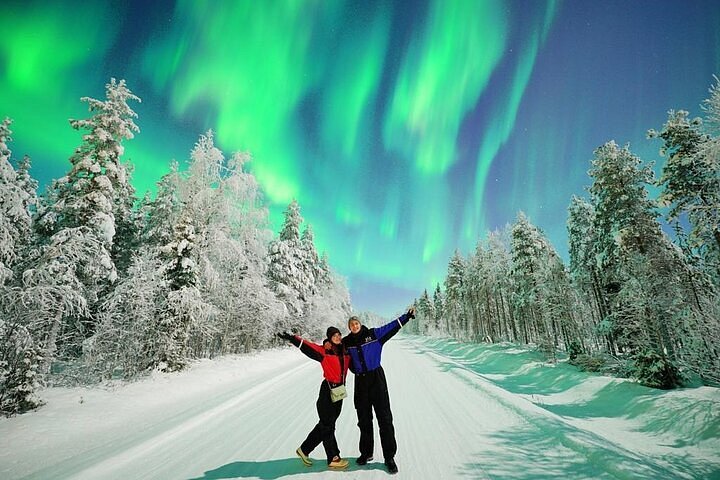In this captivating image, a couple is seen standing on a plowed, snow-covered road, surrounded by tall, snow-laden evergreen trees. The sky behind them is adorned with the mesmerizing Aurora Borealis, casting shimmering green and blue hues across the near-dusk, light sky. Positioned in the bottom center of the frame, the woman on the left is sporting a red jacket, black pants, cream-colored Air Max 97 shoes, and a white pocketbook, while the man on the right has blonde hair and is clad in a blue jacket, black pants, and black shoes. Both are dressed in heavy snow gear, complete with toboggans, and are joyfully raising their arms in the air, capturing the enchanting moment beneath nature's celestial display.